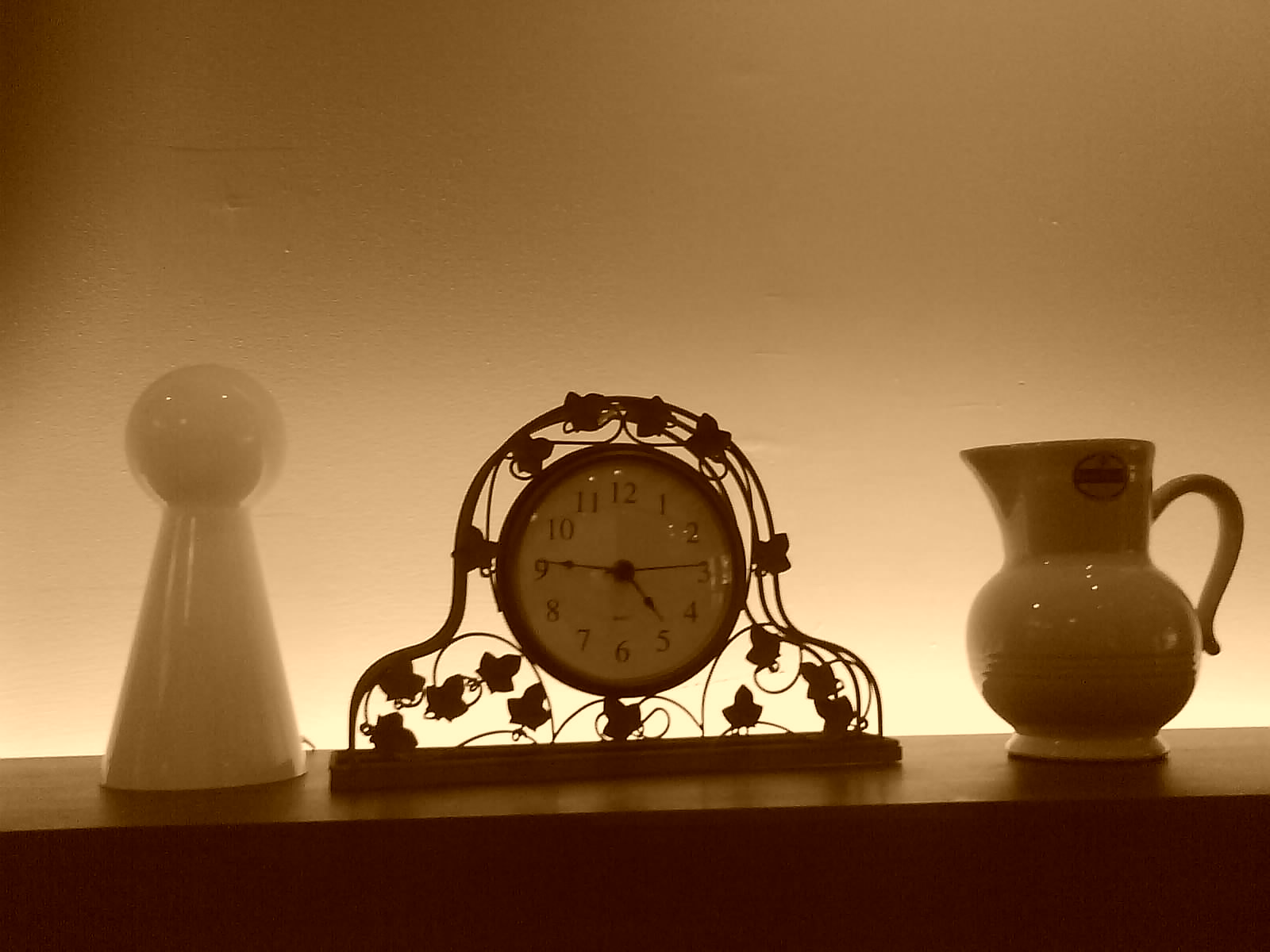This artistic photograph captures a visually captivating still life arrangement. On the left side of the image stands an intricately designed decorative ceramic object with a conical base supporting a spherical top, exuding a sense of balanced elegance. Adjacent to this ceramic piece is a round clock, featuring a white face with dark numerals and hands, encased in a metallic body decorated with a delicate, leafy floral pattern intertwined with some wires, adding an element of vintage charm. Completing the scene is a ceramic jug positioned next to the clock, distinguished by its lined details near the base. All these objects rest on a sturdy wooden shelf, which adds a rustic touch to the composition. The background reveals a light-colored wall with subtle pock marks, enhancing the texture and depth of the image. A gentle glow emanates from behind the clock, providing a warm and inviting ambiance to the overall setting.